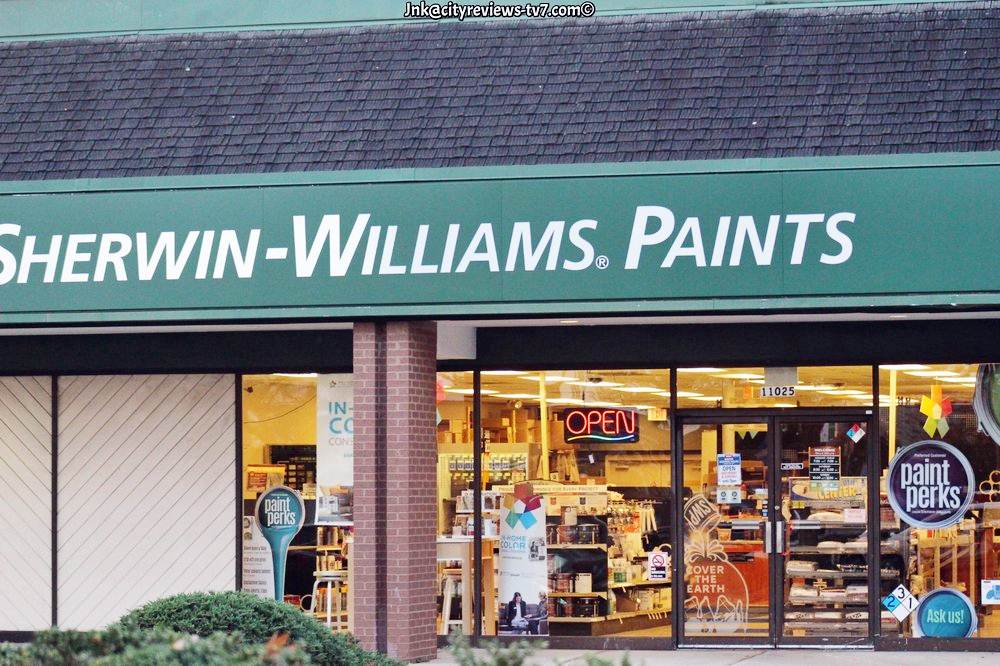This image appears to be a screenshot taken from an unspecified website, showcasing the exterior of a Sherwin-Williams Paints store. The store's name is prominently displayed on what could be described as an awning, written in white letters against a tealish-green background. The roofing is visible and is a standard black color. The upper portion of the building seems to continue the tealish-green theme, while the lower part has exterior walls that look like brown concrete. Large windows dominate the facade, including a floor-to-ceiling glass door that is partly glass and partly either wood or concrete. Through these windows, various paints and supplies are visible, and the door is adorned with several signs. An "Open" sign is also present, inviting customers in. Additionally, there is some shrubbery visible in the vicinity. At the top of the screenshot, the text "JNK at CityReviewsTB7.com" is displayed.